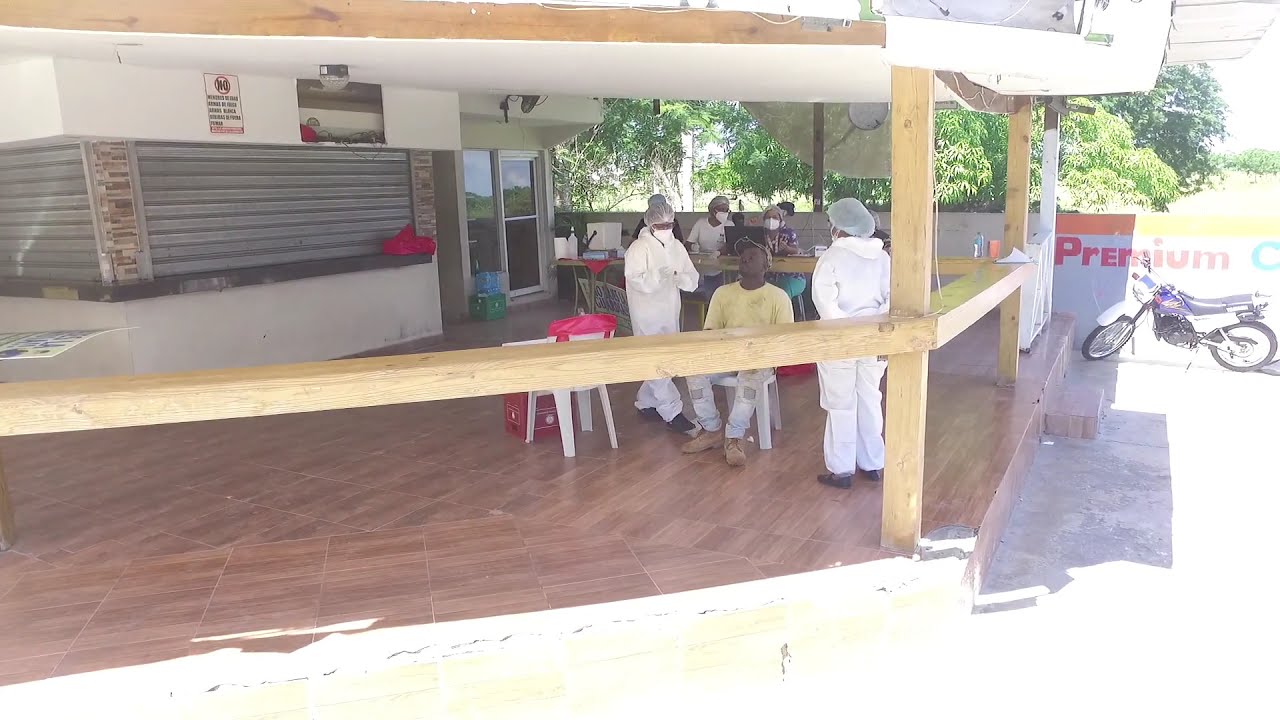This image depicts a repurposed outdoor eating area that now serves as a medical testing or vaccination site. The space features a wooden floor and is sheltered by a covered porch, with a waist-high wooden railing made up of posts and a horizontal beam. Adjoining the area is a building with an orange and yellow wall, which bears the partially visible word "premium" in red lettering and a light blue "C." There is a plastic chair where a man in light blue jeans, light brown shoes, a yellow shirt, and a hat sits, appearing to be prepared for testing or vaccination by a group of workers. These workers are dressed in white hazmat suits, complete with hairnets and masks for protection. Additional details include a closed ordering station with a lowered grate, green totes, and some red elements on nearby shelving. Further in the background, a motorcycle is parked, underscoring the multifunctional nature of the space.